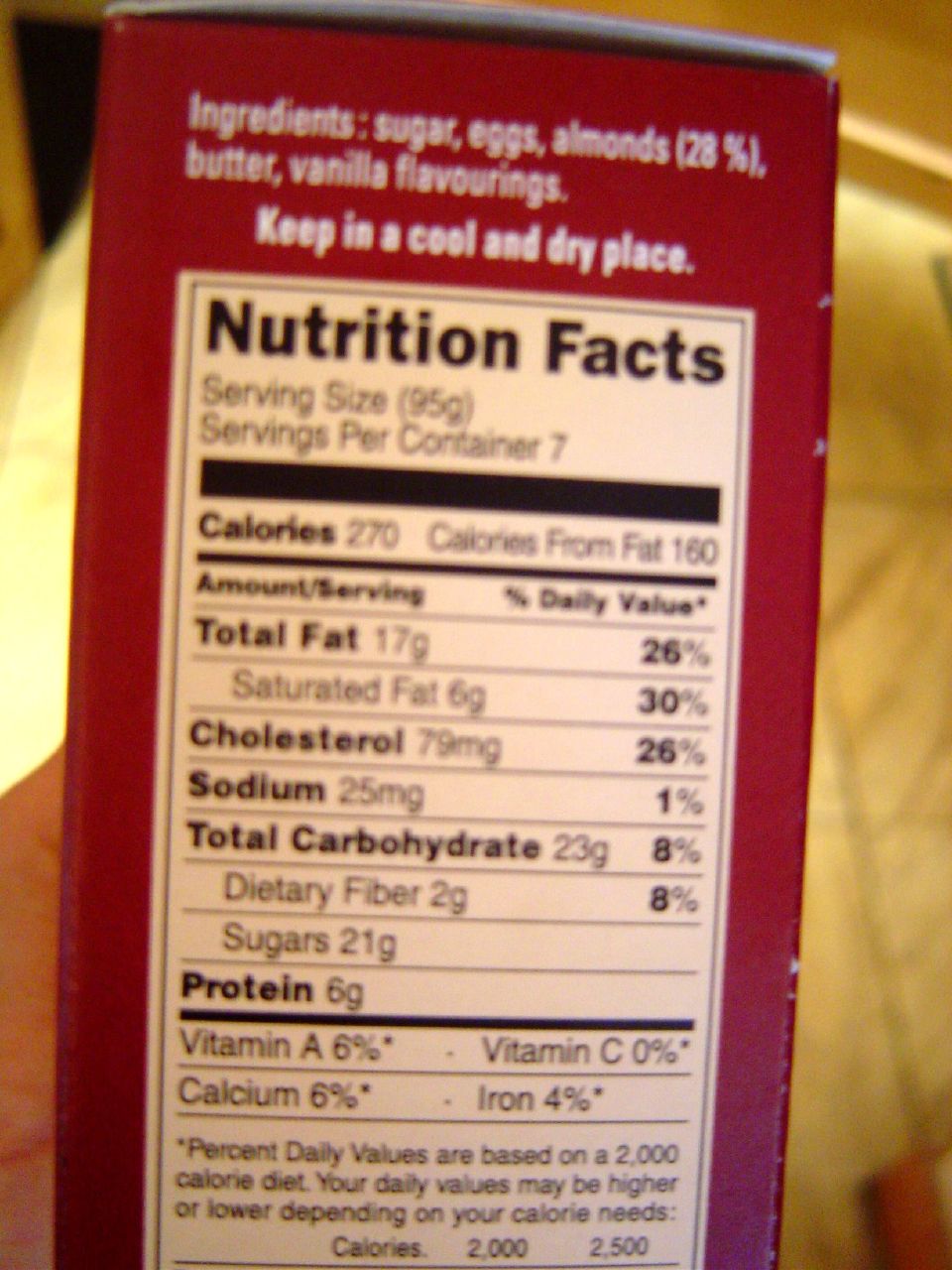This image displays the side of a dark red box, highlighting the nutrition facts label. At the top, in white font, it reads "Ingredients," followed by a list including Sugar, Eggs, Almond (28%), Butter, and Vanilla Flavorings. A note beneath advises to "Keep in a cool and dry place." Below this, enclosed in a white rectangle with a thin black border, are the Nutrition Facts. The bolded heading "Nutrition Facts" is at the top in black font. The label details serving size and servings per container, separated by a thicker black bar from the calorie information. Beneath that, separated by another thin black bar, are the measurements for fat, cholesterol, sodium, carbohydrates, and protein. The right-hand column lists the corresponding percentage daily values for each nutrient.